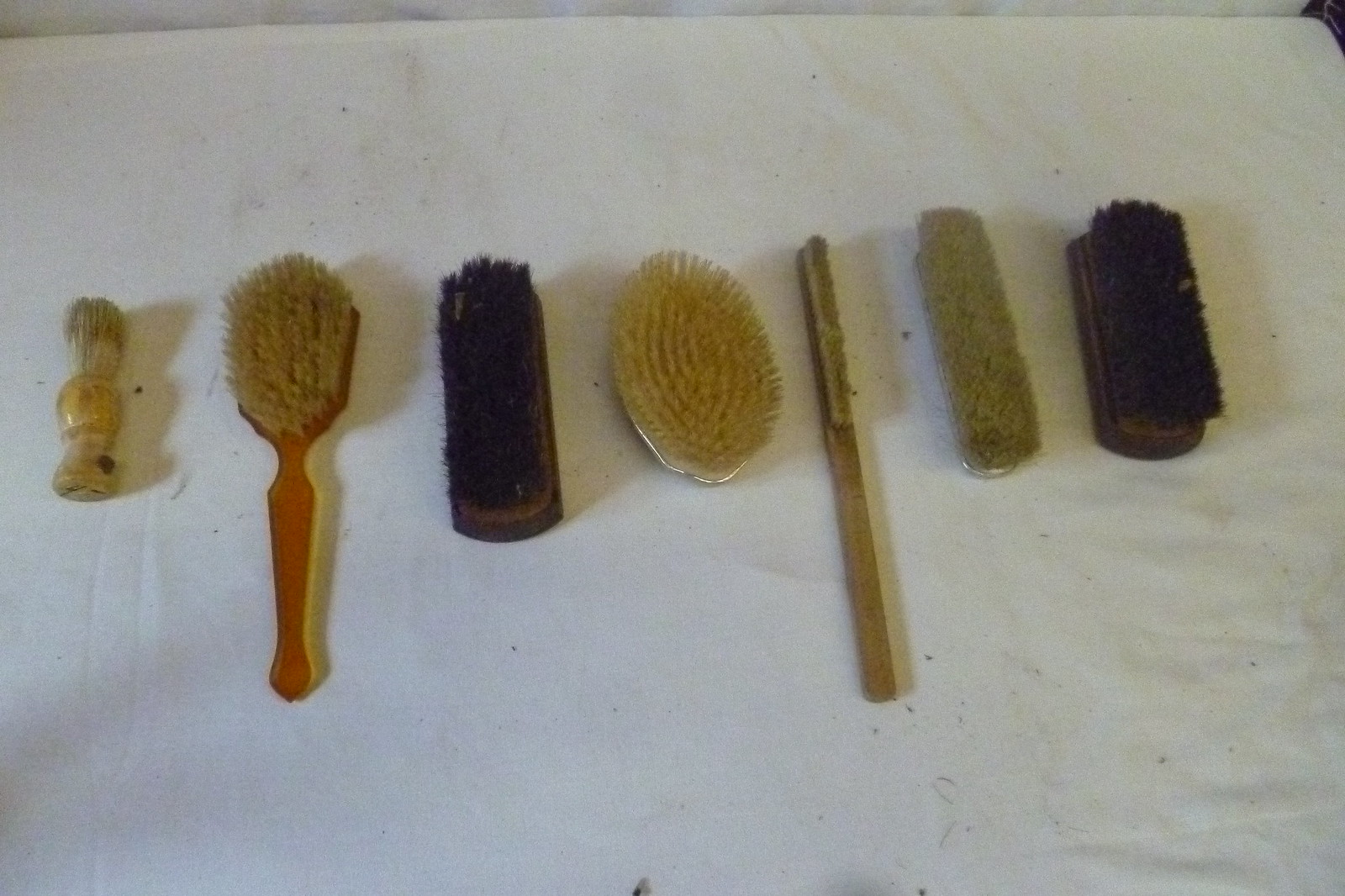The image features a collection of seven distinct brushes, meticulously arranged side-by-side on a piece of white fabric. Each brush is unique, showcasing a variety of types and potential uses. Starting from the left, the first brush appears to be a compact shaving brush with light beige bristles and an amber handle, commonly used by barbers to lather soap on the face. Next to it is a hairbrush with a long brown handle. Following that is a black-bristled brush likely used for polishing shoes or boots. The fourth brush in line is round, possibly designed for currying a horse or perhaps even a skin-massaging brush to stimulate circulation. Beside it is a hairbrush without a handle, featuring white bristles. The sixth brush is a long, slender one, possibly for cleaning narrow spaces or between cracks. Finally, the seventh brush, much like the third, appears to be another shoe polishing brush, dark in color with black bristles. The brushes' varied designs and implied functions contribute to a rich tableau of utility and craftsmanship.